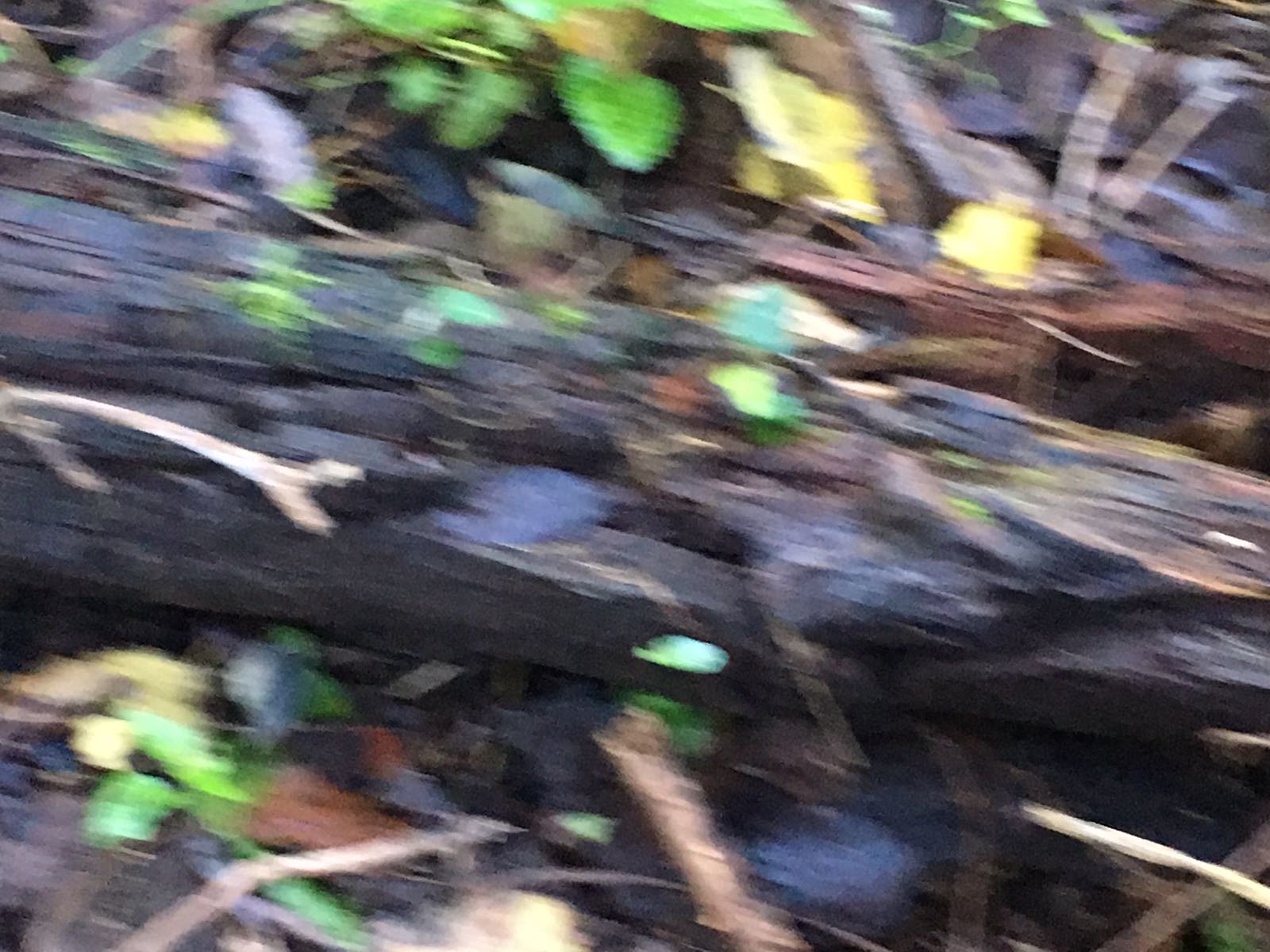This image captures a close-up view of the forest floor, presenting a somewhat blurry and highly zoomed-in perspective. It prominently features a small, almost black log, or rather a thick stick, lying horizontally across the frame from left to right. The log appears aged, suggesting it has been there for some time, and is adorned with patches of green leaves, either growing out of it or lying on its surface. Surrounding the log, the ground is littered with a mix of brown, fallen leaves and numerous smaller sticks. Additional plants can also be seen growing at the top and bottom edges of the image, contributing to the lush, layered texture of the woodland scene.